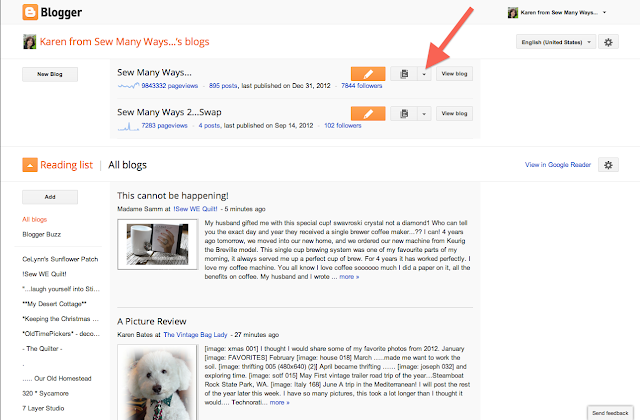This detailed screenshot captures the interface of a Blogger website page. At the top, there is a grey header where the Blogger logo is positioned on the far left. To the far right, the header displays a dropdown menu indicating the user, "Karen from So Many Ways," with a small square profile photo adjacent to the name.

The main body of the screenshot features a white background. In the upper left corner, the text "Karen from So Many Ways Blogs" appears in bold red font, with Karen's profile picture located to its left. Immediately below this heading, there is a grey button labeled "New Blog." Adjacent to this button is a grey box that reads "So Many Ways" followed by ellipses.

On the far right, an orange button displaying a white pencil icon for editing is positioned next to a dropdown box, which is highlighted by a red arrow edited into the image. Further right, there’s a box labeled "View Blog."

Below this section, the screenshot shows another blog entry following the same format with an edit button, a dropdown box, and another "View Blog" button. Beneath these entries, the text "All Blogs" is displayed, followed by a boxed preview snippet of each blog listing, providing an overview of the blog posts.

The image effectively highlights the structure and options available on Blogger’s interface, emphasizing the key functionalities and navigation elements.